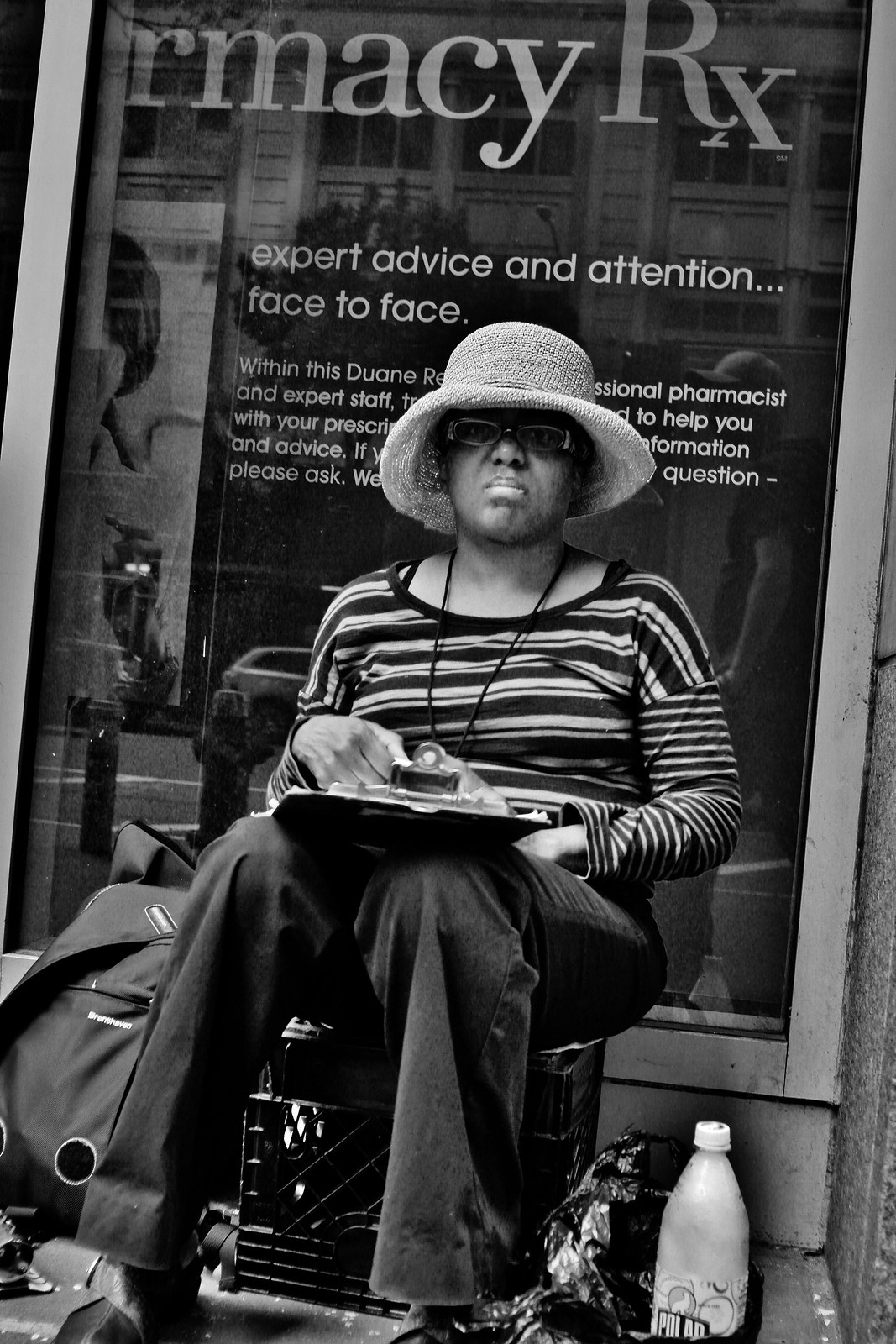In this monochromatic image, a woman is centrally positioned against a store window with the text "Armisee Rx" and "expert advice and attention face-to-face" partially visible behind her. The photograph appears to be of an older generation due to its black-and-white tones. The woman, wearing a striped long-sleeve shirt and a sun hat, sits on a plastic milk crate. She has a downcast expression and holds a clipboard on her lap, with a book bag to her left and a bottle partially concealed in a plastic bag beside her on the ground. The setting exudes a daytime outdoor atmosphere, with various objects like bags and bottles scattered around, suggesting she might be experiencing homelessness.